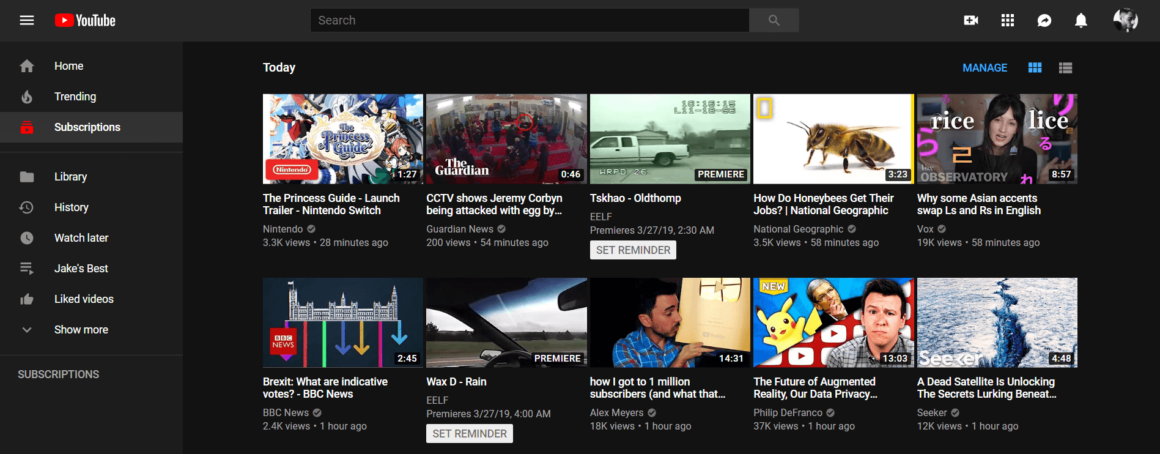The image captures a YouTube page with the predominant background being black. At the top of the screen, the iconic YouTube symbol, a red rectangle with a white play button, is distinctly visible. On the left sidebar, various navigation options are listed, each accompanied by respective icons. The "Home" option features a house icon, "Trending" is marked by a fire icon, and "Subscriptions" is highlighted in red, denoted by a folder icon. Below these, the "Library" section displays a folder, "History" is represented with a refreshing icon, and "Watch Later" is indicated by a clock icon. Additional options like "Jake’s Best" (three lines icon), "Liked Videos" (thumbs up icon), and "Show More" (arrow down) are also detailed. The "Subscriptions" segment follows these icons.

The main page showcases a series of video thumbnails. At the top, five videos are displayed under the "Today" label, and another set of five videos is listed below them. Each video thumbnail includes a preview image along with the video’s duration in minutes and seconds. For instance, notable videos are "The Princess Guide Launch Trailer" associated with the Nintendo Switch, "The Guardian OOC: Jerry Corbin Attacked with Eggs," "Tahashqo Old Dump," and "How Do Honeybees Get Their Jobs?" among others. The timestamps of when the videos were uploaded are also visibly marked.

This depiction provides a comprehensive view of the YouTube platform interface, showcasing both the navigational elements on the left and the recommended video content in the central section.